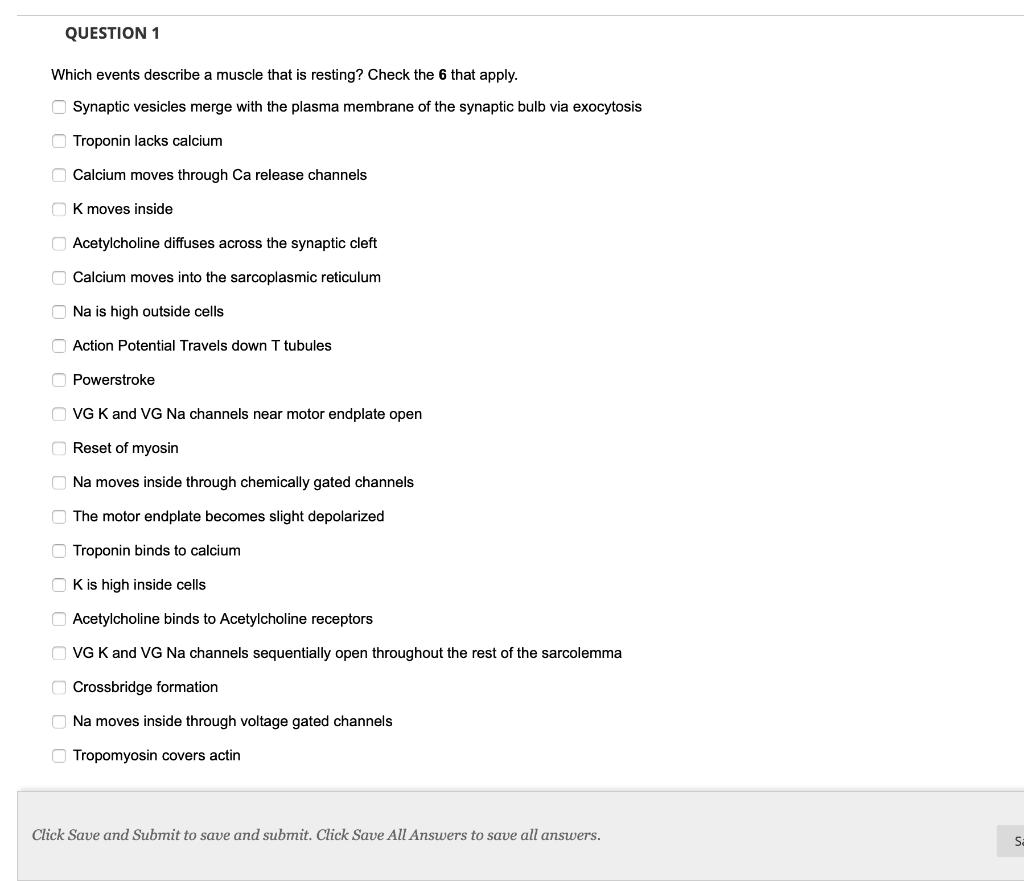The screen displays a lengthy list of events associated with muscle physiology. The primary prompt asks, "Which events describe a muscle that is resting? Check the six that apply." The list includes technical terms such as "Calcium moves through CA release channels," "Potassium (K) moves inside," "Calcium moves into the sarcoplasmic reticulum," "Sodium (NA) is high outside the cells," and "Reset of myosin." The complexity of the terminology is evident, indicating that the subject matter is advanced. Below this list, there is a single bar with options to "Save and Submit" or "Save All Answers."